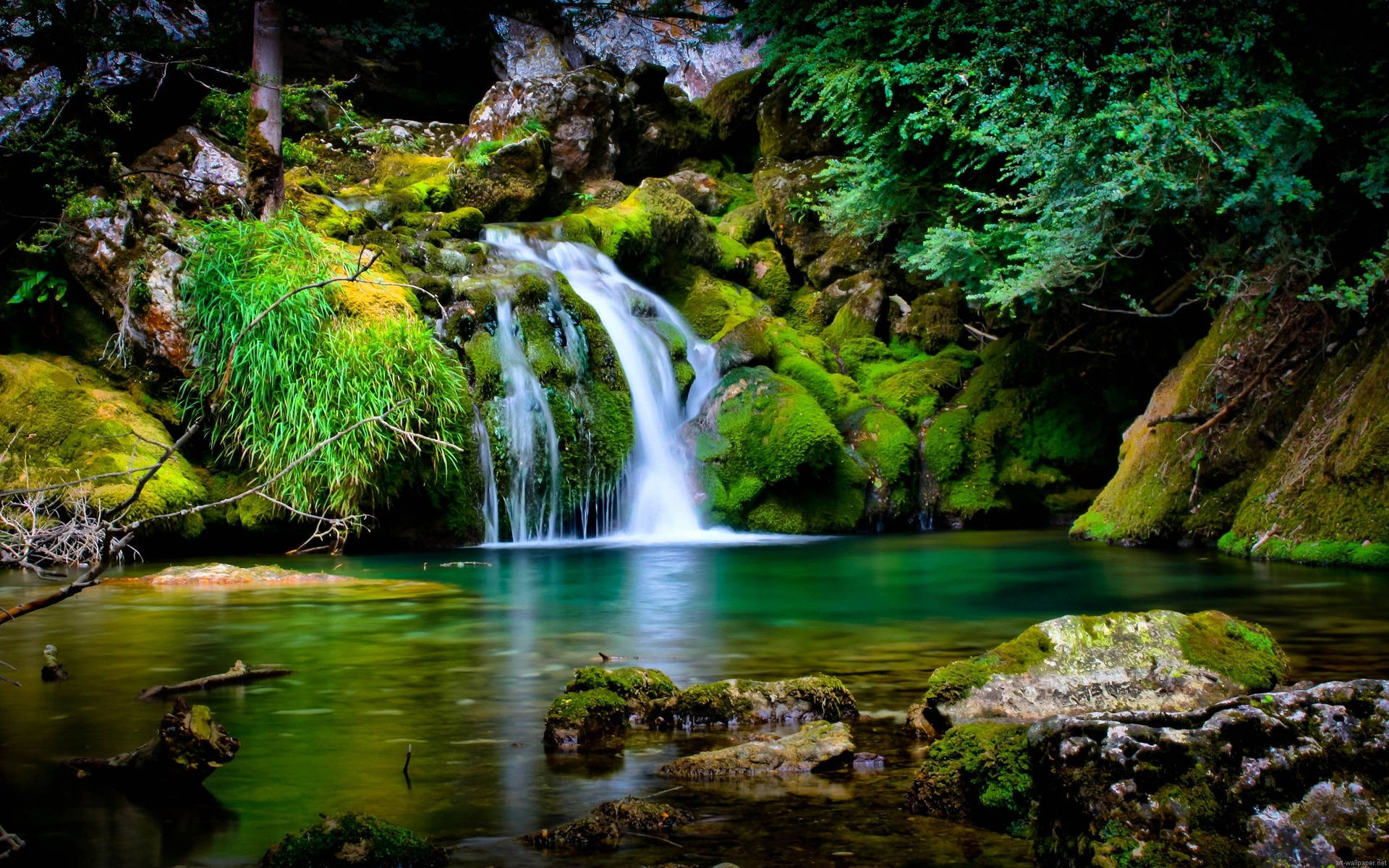This highly detailed and tremendously vibrant depiction of a serene natural scene appears almost surreal due to its intense coloration and saturation. Dominated by lush green hues, the image showcases a small, picturesque waterfall gracefully cascading over moss-covered rocks into a tranquil river or pond. The water appears strikingly blue, contrasting beautifully with the surrounding greenery. Moss blankets the rocks, creating a lush, textured look that almost begs to be touched. The scene is peppered with various trees and tree branches, including a prominent cedar and a tall tree trunk extending from the top of the image. The overall effect is one of an ethereal, art-like quality, with colors so vivid and bright they suggest either a high-resolution photograph or a digitally enhanced painting. The combination of the flowing water, rich green moss, and detailed foliage makes this image exceptionally relaxing and visually captivating.